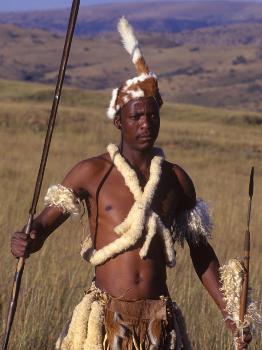The photograph captures a black indigenous man standing in a vast green grassy field with rolling hills and distant mountains in the background. He is adorned in tribal attire, including a distinctive brown and white cowhide headdress with a cow tail protruding from it. His chest is crossed by a white fuzzy cylindrical scarf-like object that wraps around his neck and shoulders, creating an X shape. He wears matching white bands immediately below his armpits on both arms, and his waist is draped in a brown skirt accented with more white animal hide. In his left hand, he holds a short spear-like weapon with white wooly frills, while his right hand grasps a much longer spear. The detailed backdrop and traditional attire together create a powerful image of cultural heritage and the natural environment.